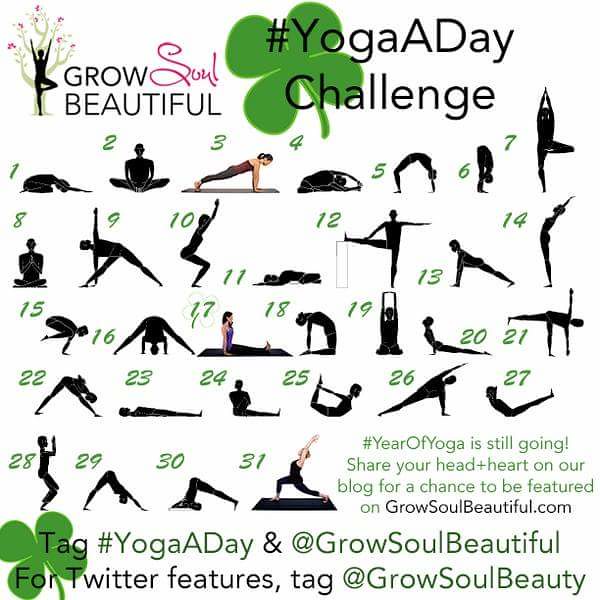The image features a white background dominated by the black silhouettes of 31 different yoga poses, each corresponding to a day of the month. In the upper-left corner, there's a black outline of a woman practicing yoga in front of a tree with the text "Go Beautiful S-A-O-U-L." Nearby, a green four-leaf clover bears the inscription "#YogaDayChallenge." The poses range from a woman kneeling bent over on the 1st day, to another bending backward in an arch on the 5th day, and a woman standing on one leg with her left leg bent at a 90-degree angle on the 7th day. Below these silhouettes, a few poses are highlighted in full color, such as a woman in black tights and a red top. In the lower right-hand corner, the image reads, "Year of the Yoga is still going" along with a call to "Share your head and heart on our blog for a chance to be featured on GrowSoulBeautiful.com." Along the bottom, overlaid on a shamrock, there's another reminder to tag "#YogaDay" and "@GrowSoulBeauty" for a feature on Twitter, emphasizing the 31-day yoga challenge.